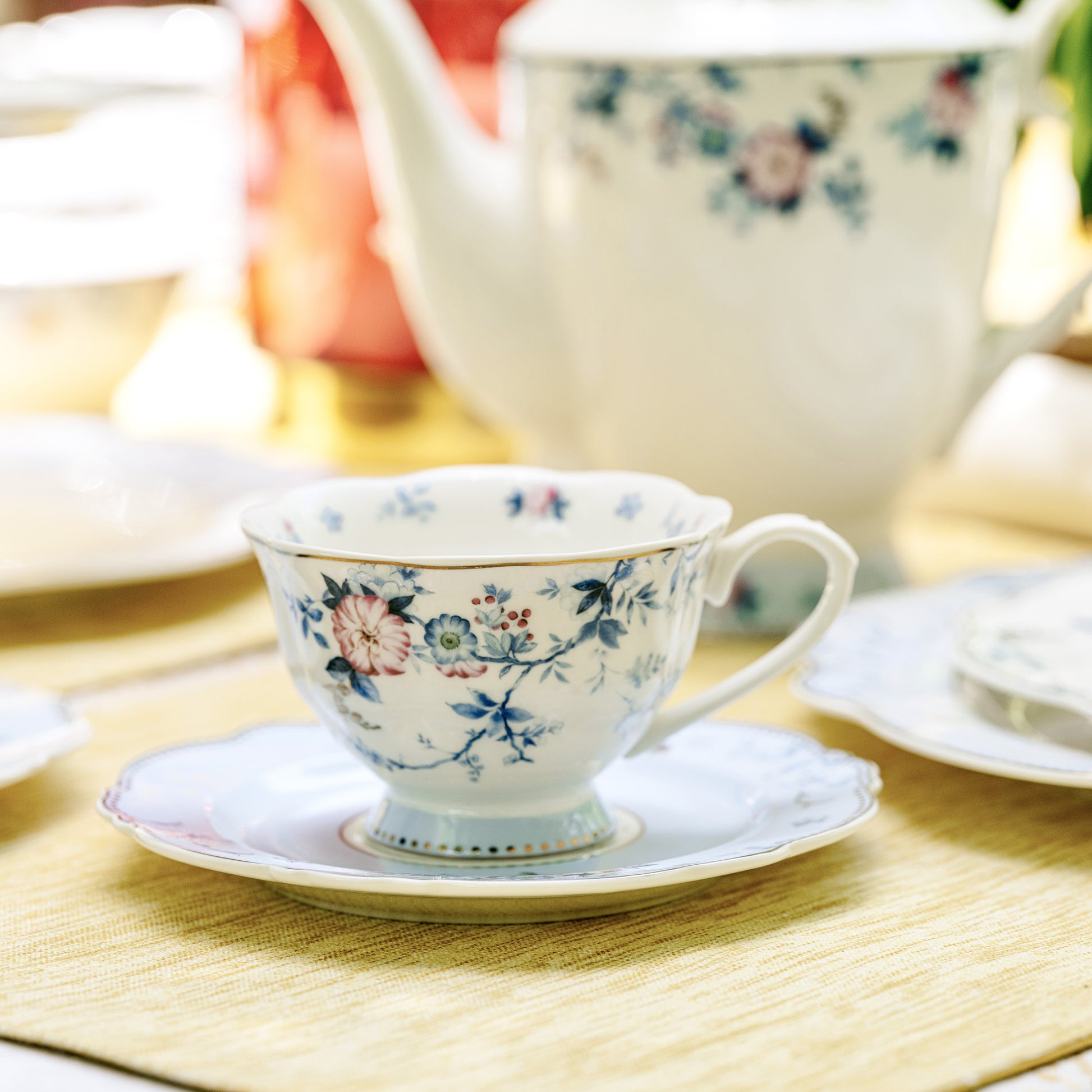This close-up image captures a delicate, old-fashioned teacup or coffee cup resting on a matching saucer. The focal point of the image is the small white china cup, adorned with intricate pink and blue flowers intertwined with blue stems, gracefully painted in a curvy pattern. The cup features a thin, elegant design with gold trim along both the upper and lower rims. The saucer, painted a pale blue, also bears a luxurious gold accent around its edges and showcases a curvaceous, floral trim.

In the background, blurred yet distinguishable, is a classic white ceramic teapot embellished with similar floral patterns, resting on a light brown wooden placemat. Additional cups and saucers, echoing the central design, are arranged nearby, creating a comforting and cohesive tea setting. The light wooden table beneath adds warmth to the scene, enhancing the vintage charm of the delicate china on display.